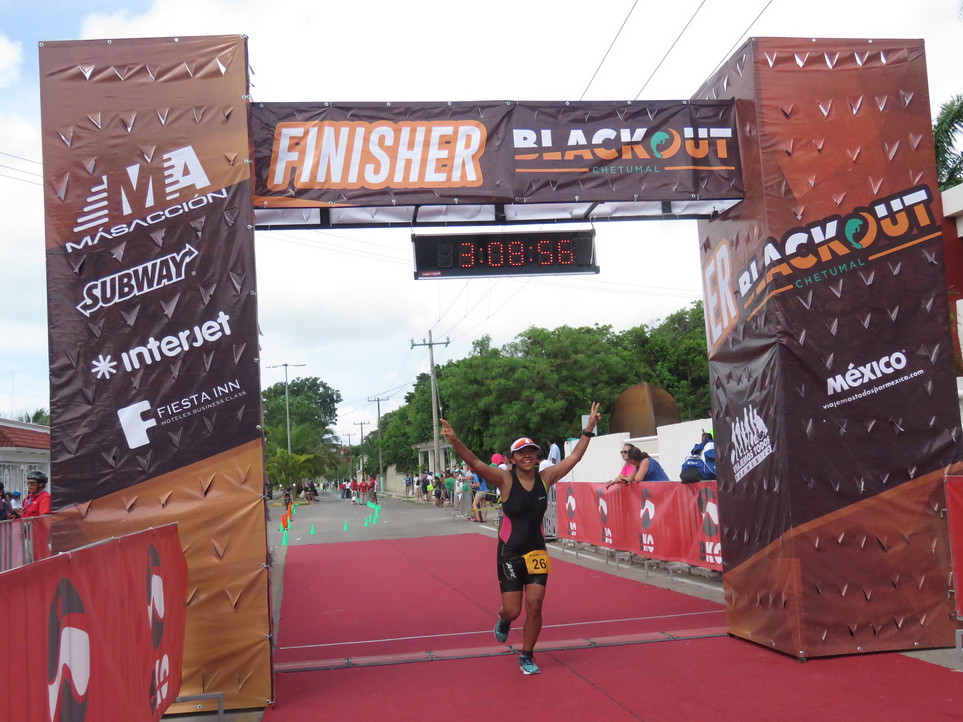The image captures the celebratory moment at the finish line of the "Finisher Blackout" road race, likely a marathon held in Chetumal, Mexico. A jubilant young woman, identifiable by her dark skin and bright white cap, crosses the finish line with arms outstretched, making V for victory signs with both hands. Her athletic outfit consists of a sleeveless, black form-fitting tunic and tight black shorts. She proudly displays a yellow number "26" on her hip. A broad smile lights up her face as the timer above her displays 3:08:56. She stands beneath a large banner adorned with advertisements from sponsors such as Masacion, Subway, Interjet, and Fiesta Inn. The finish line itself is marked by a red carpet or marking on the roadway, contrasting with her black uniform and the green pylons in the background. A few spectators can be seen lingering, observing the runners still approaching. The festive poles and banners create a vibrant atmosphere, celebrating the completion of this local marathon event.